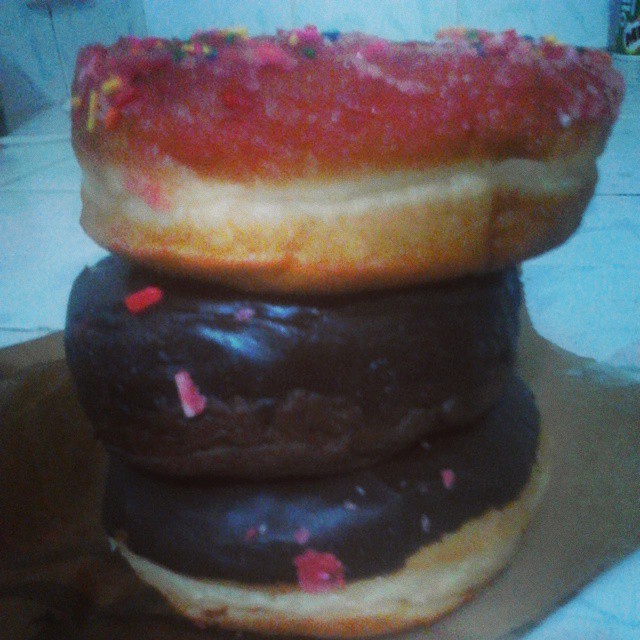The image portrays a close-up shot of three donuts carefully stacked on top of each other. The top donut features a strawberry-flavored glaze, discernible by its reddish-pink hue and an assortment of colorful sprinkles—yellow, red, green, and blue—that embellish its surface. The middle donut boasts a rich chocolate glaze, with stray sprinkles from the top donut dotting its surface. The bottom donut has a chocolate frosted top and a plain brown base, with evidence of pink glaze dripping down from the upper donuts. The entire stack rests on a medium brown paper bag, all set against a tiled floor backdrop. The image quality is quite grainy and low resolution, with a noticeable blue tint and glare affecting the overall clarity.